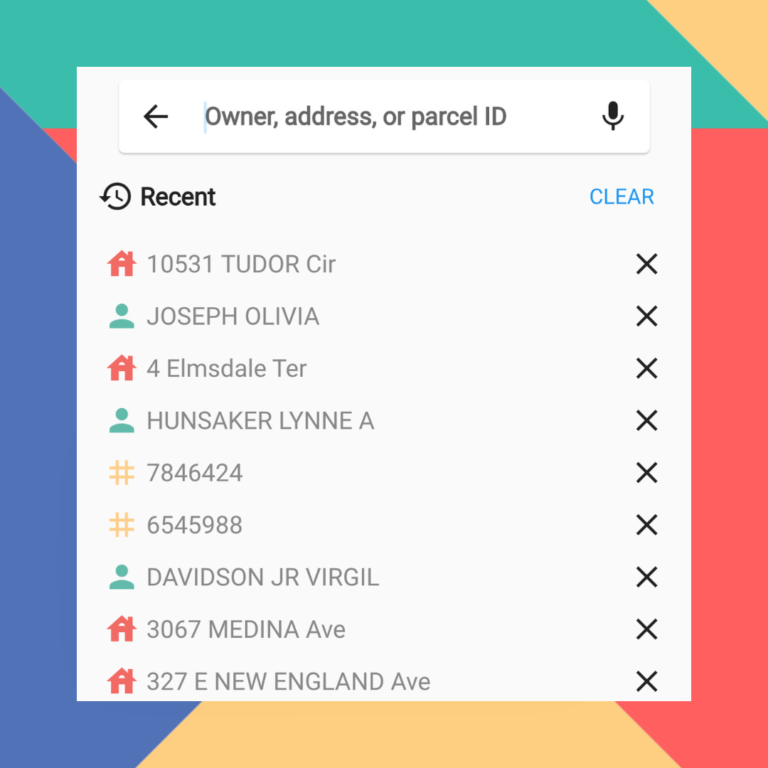The image displays a screenshot of what seems to be an application interface. The screen features a colorful geometric border in yellow, red, green, and blue, which gracefully curbs around a central white rectangular area. Within this white box, another smaller box is superimposed, creating a visual effect of a framed border. This smaller box contains the text "Owner Address or Parcel ID" and is flanked by an arrow icon on the left and a microphone icon on the right, resembling a search bar.

Directly below this search bar is a heading labeled "Recent," accompanied by a familiar icon for accessing recent activities on the left side. Aligning with the heading on the right side, the word "Clear" is prominently displayed in blue text, standing out against the otherwise uniform color scheme.

Beneath the "Recent" heading, a list of addresses and names — presumably recent entries or searches — is displayed. Examples from this list include "10531 Tudor Circle," "Joseph Olivia," and "4 Elmsdale Terrace." The list contains around ten entries, concluding with "327 East New England Avenue." The screen then transitions into a simple bottom border, neatly framing the content above.